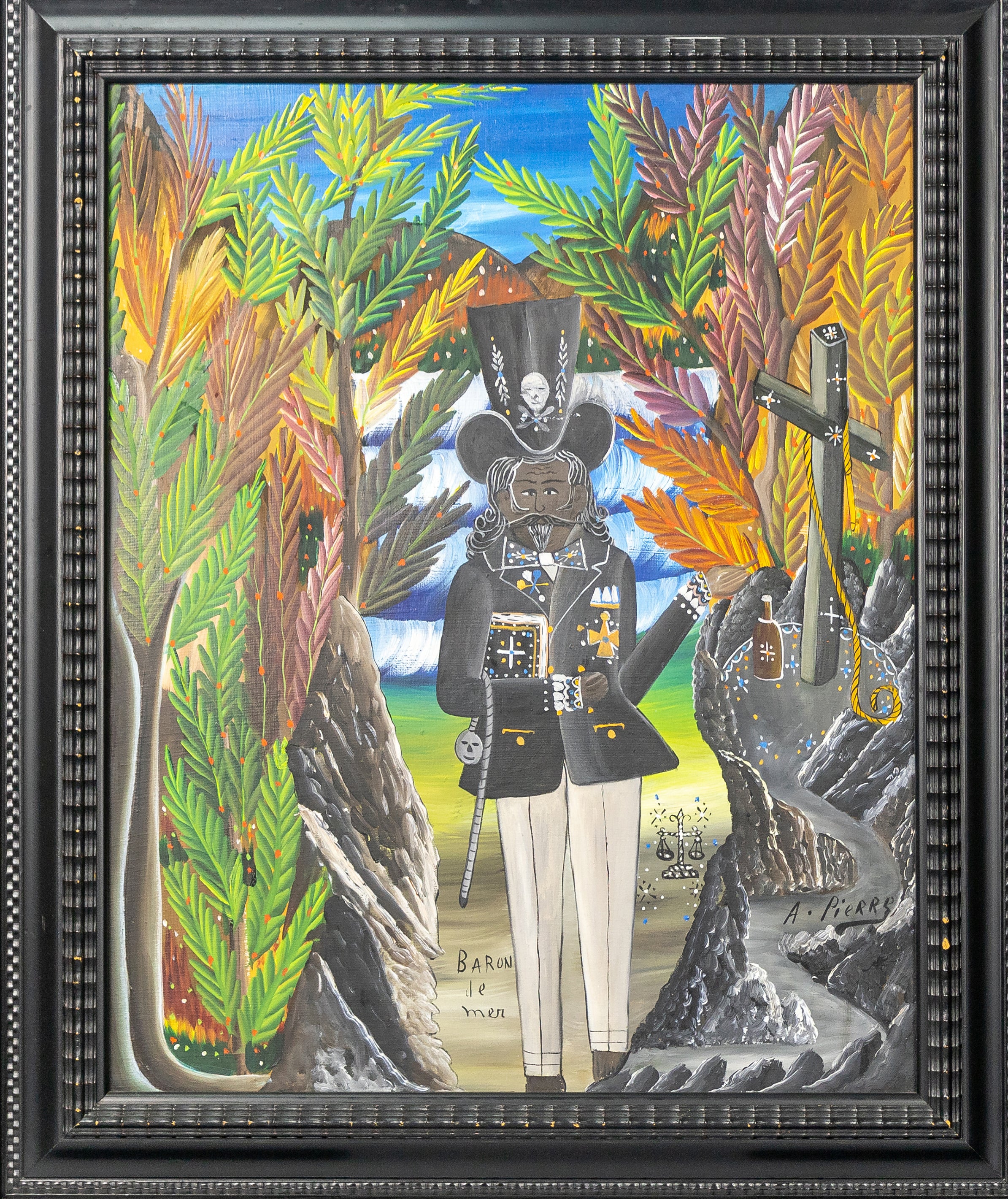The image features a framed painting displayed within a black frame adorned with small white squares. The central figure in the painting is an African-American man with dark brown skin, donning a black jacket with cross-like patterns, a black cap adorned with a skull-like design, and white pants. The man has a dark mustache and holds a book in his right hand, along with a rope-like object. Encircling him are green, maroon, and orange leaves against a vibrant blue sky. To the right of the figure are a rock-like structure topped with a cross entwined with a yellow rope and a nearby brown bottle. The left side displays a backdrop of trees and additional rock formations. In the background, there are mountains and a blue and white water-like surface. Near the bottom right is the artist's signature resembling a pear, while the bottom center contains the text "barren beamer," both inscribed in black.